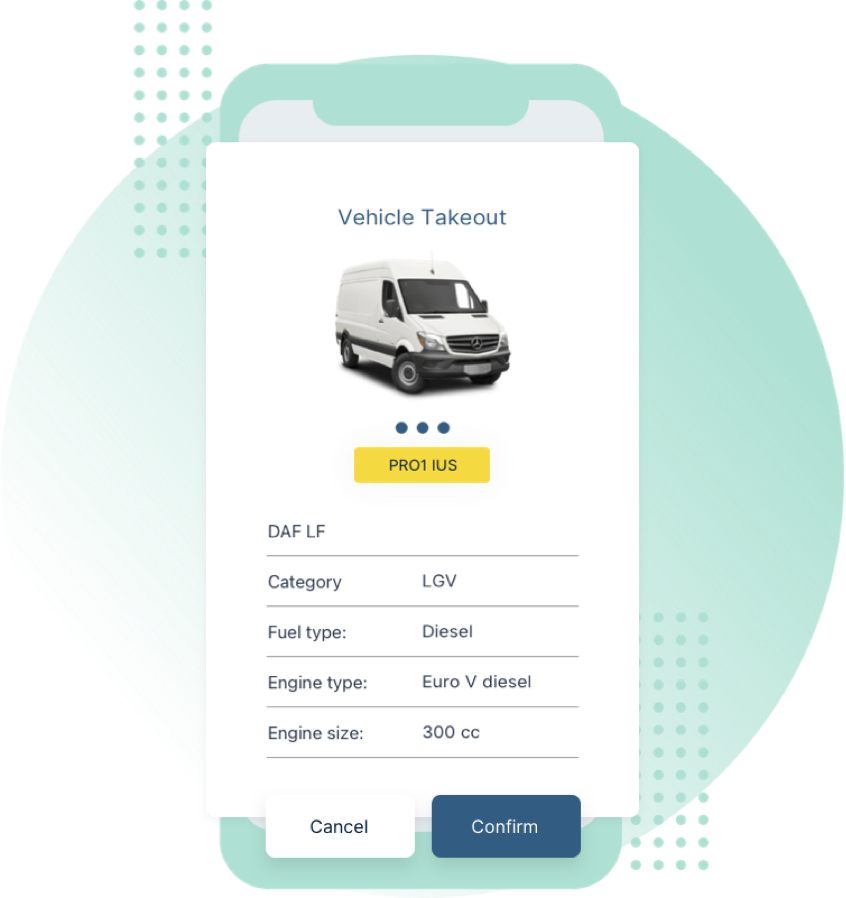The image is a detailed screenshot of an interface displaying a vehicle profile, specifically a white van. At the top of the interface, the title "Vehicle Takeout" is prominently displayed in blue. Directly below this title is an image of the white van. Beneath the van image are three blue dots, presumably indicating additional images or details that can be viewed. Further down, a yellow button labeled "Pro 1 IUS" is centered on the screen. Below this button, descriptive text lists various specifications of the vehicle: "Category: LGV, Fuel Type: Diesel, Engine Type: Euro V Diesel, Engine Size: 3000 cc." At the bottom, the interface offers two action buttons, with "Cancel" located on the left and "Confirm" on the right, allowing users to either discard or confirm the information presented.